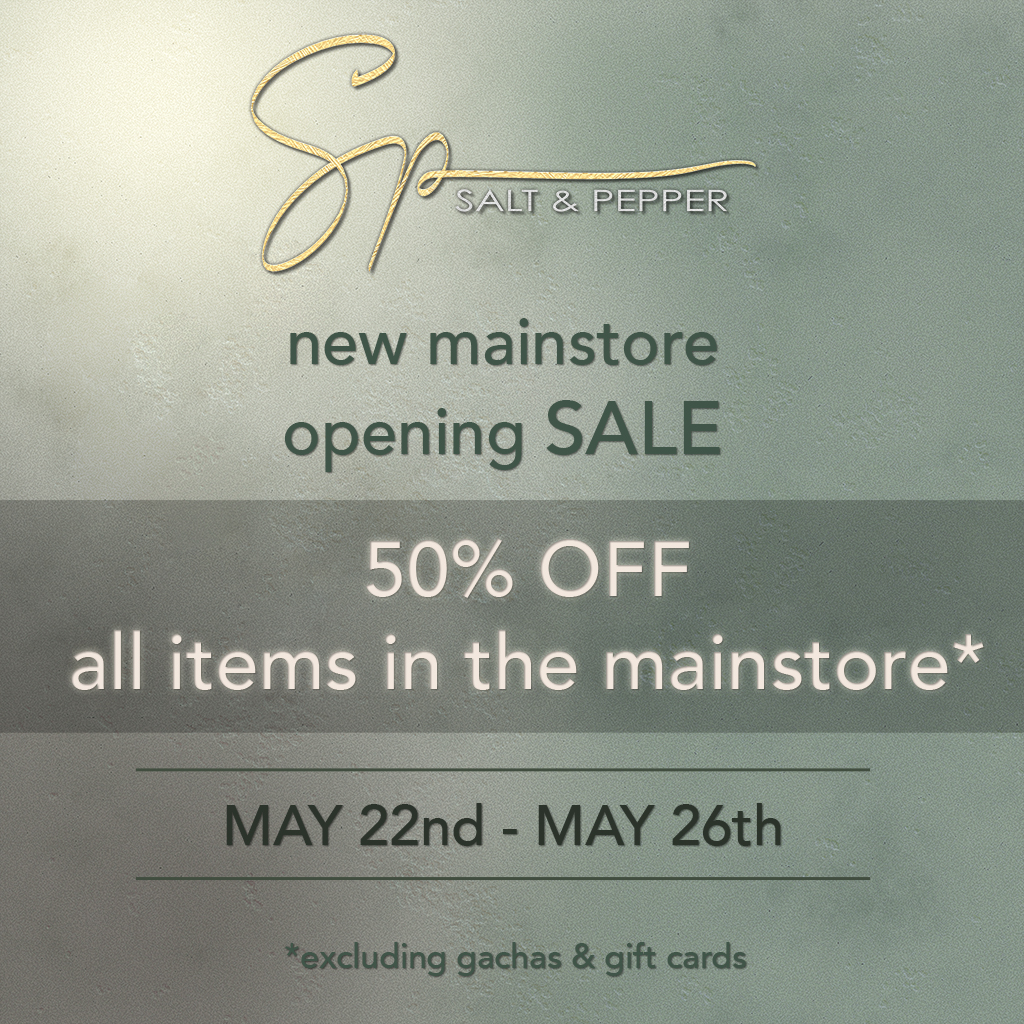The image depicts an advertisement for an SP Salt and Pepper store, showcasing their new main store's opening sale. The advertisement, which could be a poster or banner, features a background with a gradient of light to darker army green, mimicking the look of a wall. At the top, the store's logo, a gold-colored "SP," stands out, followed by the name "Salt and Pepper" in white lettering. The prominent announcement, "New Main Store Opening Sale," is highlighted with the word "SALE" in bold, uppercase green letters. Beneath this, a dark green horizontal strip contains the offer: "50% OFF all items in the main store," written in white lettering. An asterisk following this text points to a footnote at the bottom of the image that reads, "excluding gachas and gift cards." The sale is scheduled for May 22nd to May 26th, with these dates enclosed in borders made by black lines. There are no people depicted in the image, emphasizing the banner's straightforward promotional message.